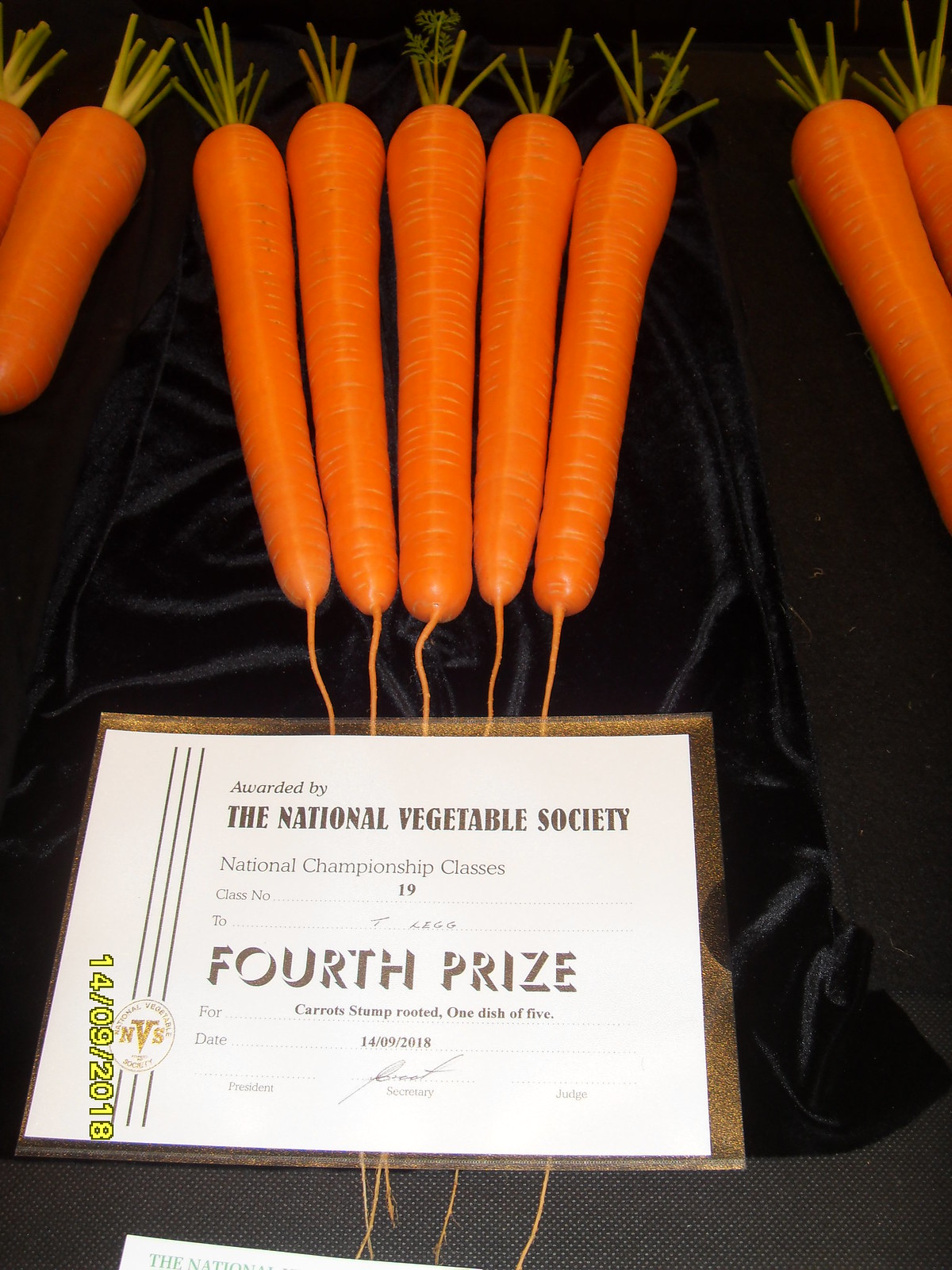A tall rectangular image depicts a bundle of five exceptionally large and bright orange carrots arranged neatly on a table. The dark gray tabletop is elegantly draped with a silky, velvety black cloth. Each carrot points downwards and showcases short, green, trimmed sprouts at the top. Flanking this central bundle are the edges of other carrot bundles. 

At the bottom of the image, partially covering the velvety cloth, lies a white laminated certificate with a gold trim, awarded by the National Vegetable Society. The certificate is printed in black and dark brown fonts, stating: "National Championship Classes, Class Number 19, Awarded to T. Legg. Fourth Prize for Carrot Stump Rooted, One Dish of Five. Date: 14-09-2018." The certificate bears a signature at the bottom, adding to the sense of official recognition for these carefully presented vegetables.